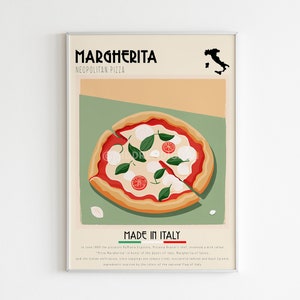This is an image of a rectangular poster framed by a thin silver metal frame, set against a pure white background. The poster itself features a beige-colored background and displays the word "Margarita" in an all-caps, Art Deco font at the top left. To the right, there is a black silhouette of the country of Italy. Beneath this, a cartoon image of a pizza dominates the center; it's depicted with a circular shape, cut diagonally. The pizza showcases melted mozzarella cheese, scattered basil leaves, and slices of tomatoes, all atop red marinara sauce, which edges the light beige crust. At the bottom, the poster states "Made in Italy," followed by a thin rectangular depiction of the Italian flag in green, white, and red. There is additional, barely legible text beneath this, blending into the background.